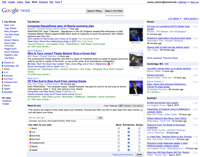The image is a screenshot from a website, displayed in landscape orientation suitable for a laptop or computer monitor. The background is white and the screenshot is very blurry, making it difficult to read any text clearly. The layout is divided into three columns. 

The left column is narrower and contains a menu with blue text links. This menu features color-coded indicators, such as rectangles or dots, in various colors next to the options. The colors include blue, green, yellow, gray, red, and another yellow and blue. These may represent different categories or statuses of the menu items.

The middle column is the main content area. It contains both black and blue text, with the blue text presumably representing clickable links. Square photographic thumbnail images are also present alongside the text, suggesting that each item may be a news article with accompanying multimedia.

The right column appears to house additional clickable articles or links, though the specific heading is unclear due to the blurriness. This column may serve as a supplementary navigation area for related content.

Notably, the top-left corner of the screen displays the Google News logo, although the word "news" is in lowercase and hard to decipher clearly. Next to the logo, there is a search bar.

Overall, despite the blurriness, the layout and elements suggest that this is a screenshot of the Google News website, featuring a main content column with news stories and additional navigation or related articles on the sides.